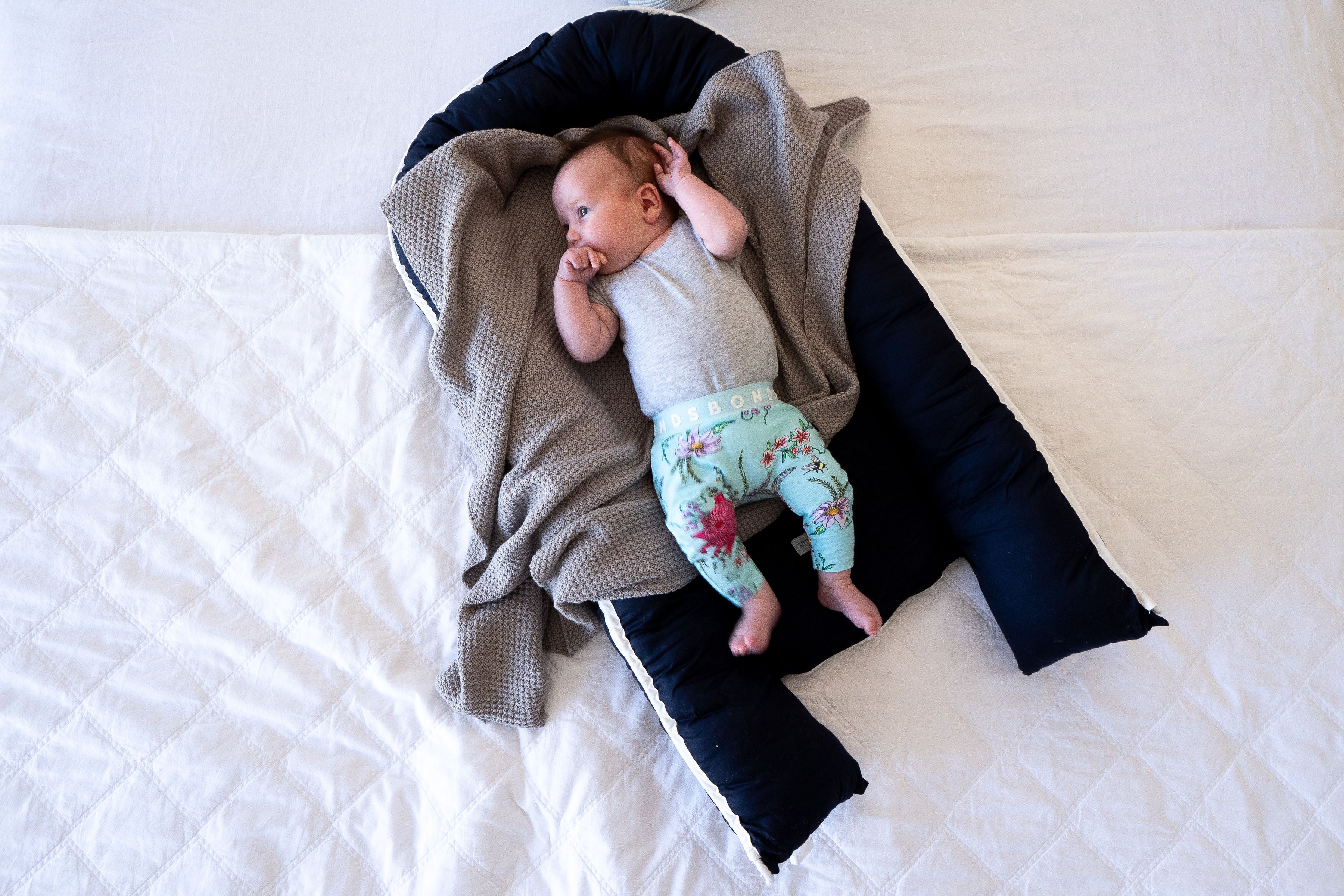In the photograph, an infant is nestled in a cozy, rounded, and oblong black cushion or soft bed. The cushion is adorned with a gray, knit blanket, upon which the baby comfortably lies. The infant is dressed in a gray t-shirt and green pants patterned with flowers. Its head is turned to the side, and it appears to be chewing on its right hand while the other hand is raised in the air. The entire setup is placed atop a white, soft surface, likely the middle of a large bed, though the edges of the bed are not visible. The scene captures the serene, innocent moment without any accompanying text.